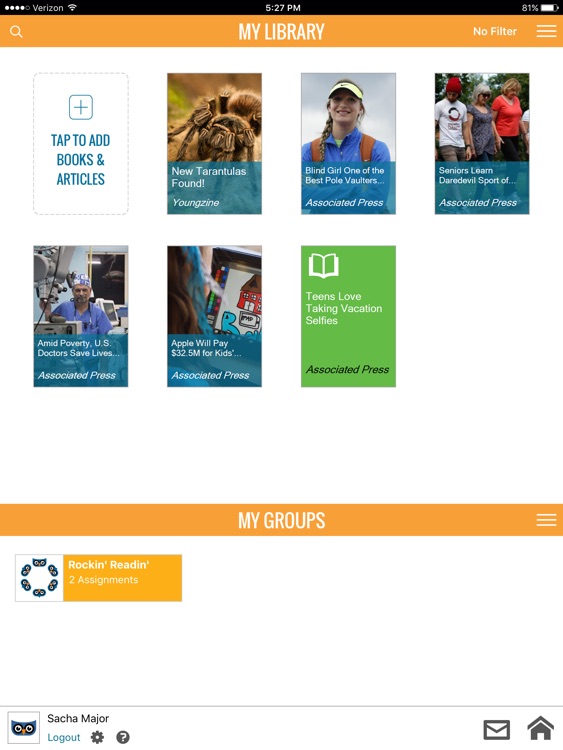In this detailed image description, a smartphone displaying a website is shown openly. The smartphone screen displays the current time as 5:27 PM, an 81% battery life, and both a network signal icon and a Wi-Fi icon. The service provider is Verizon. 

The website's header has an orange background with white text bearing the title "My Library." To the right, there's a "No Filter" label and a menu icon represented by three horizontal lines. On the left side of the header, a search bar icon is visible.

The webpage's main content area has a white background and exhibits six books at the center. The first prompt invites the user to "Tap to add books and articles," with "Add Articles" written in blue text. The showcased books include:

1. **New Tarantula Found** by Yang Xin.
2. **Planned Care** by one of the best-polled vouchers from the Associated Press.
3. **Seniors Learn Daredevil Sports Amid Poverty**.
4. **U.S. Doctors Save Lives**.
5. **Apple Will Pay $32.5M for Kids**.
6. **Teens Love Seeking Vacation Selfies**, which is green in color.

At the bottom of the page, a text box labeled "My Groups" is present, set against an orange background. On the bottom left, an option titled "Rocking Reading to Assignment" also appears on an orange background. Further down on the left-hand corner, there is an area labeled "Search Major Logout," accompanied by an image of an owl colored in blue, black, and yellow.

In the bottom right corner of the page, two icons are displayed for email and home navigation.